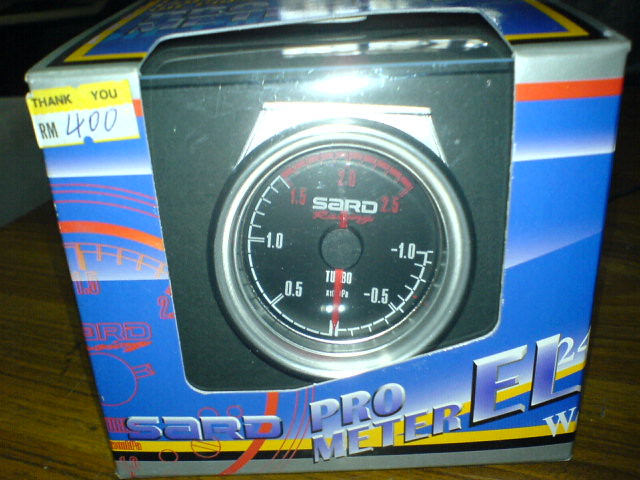This photograph showcases a packaged electronic device designed for sale. The packaging is predominantly blue with a sophisticated design featuring a red dial illustration. At the bottom of the box, the text "SARD PROMETER L" is prominently displayed. A clear plastic window on the front reveals the product inside.

The device itself is a sleek black box with a prominent circular dial on the front. The dial is encased in a silver frame, with a black face dotted with numerals. The white and red numerals appear as follows: starting at -1, then -5, -0.5, 0.5, 1.0, and in red: 1.5, 2.0, and 2.5. The dial also features the branding "SARD" in white, and beneath it, a word written in red cursive. At the dial's base, the words "WHITE TURBO" are inscribed.

Additionally, a sticker with a yellow "THANK YOU" message and an "RM400" price tag on a white background are attached to the device. The entire boxed unit is positioned on a wooden surface.